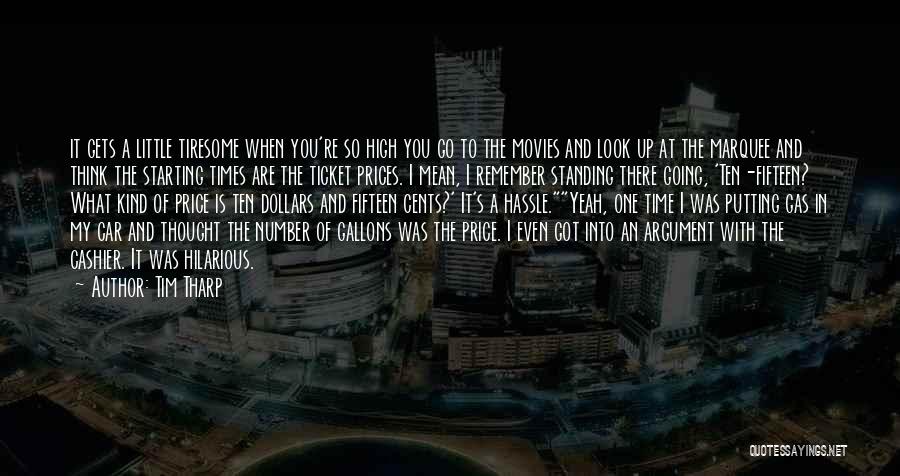In the dimly-lit image, a sprawling cityscape unfolds beneath a dark night sky, vibrant with the myriad lights of skyscrapers and street lamps. Superimposed in bold white capital letters at the center of the image is a quote by Tim Tharp, though the author's name appears slightly blurry. The quote humorously recounts, "It gets a little tiresome when you're so high you go to the movies and look up at the marquee and think the starting times are the ticket prices. I mean, I remember standing there going, $10.15? What kind of price is $10.15 to hassle? Yeah, one time I was putting gas in my car and thought the number of gallons was the price. I even got into an argument with the cashier. It was hilarious." At the bottom right, a watermark reads "QuotesSayings.net," affirming the source of the image.